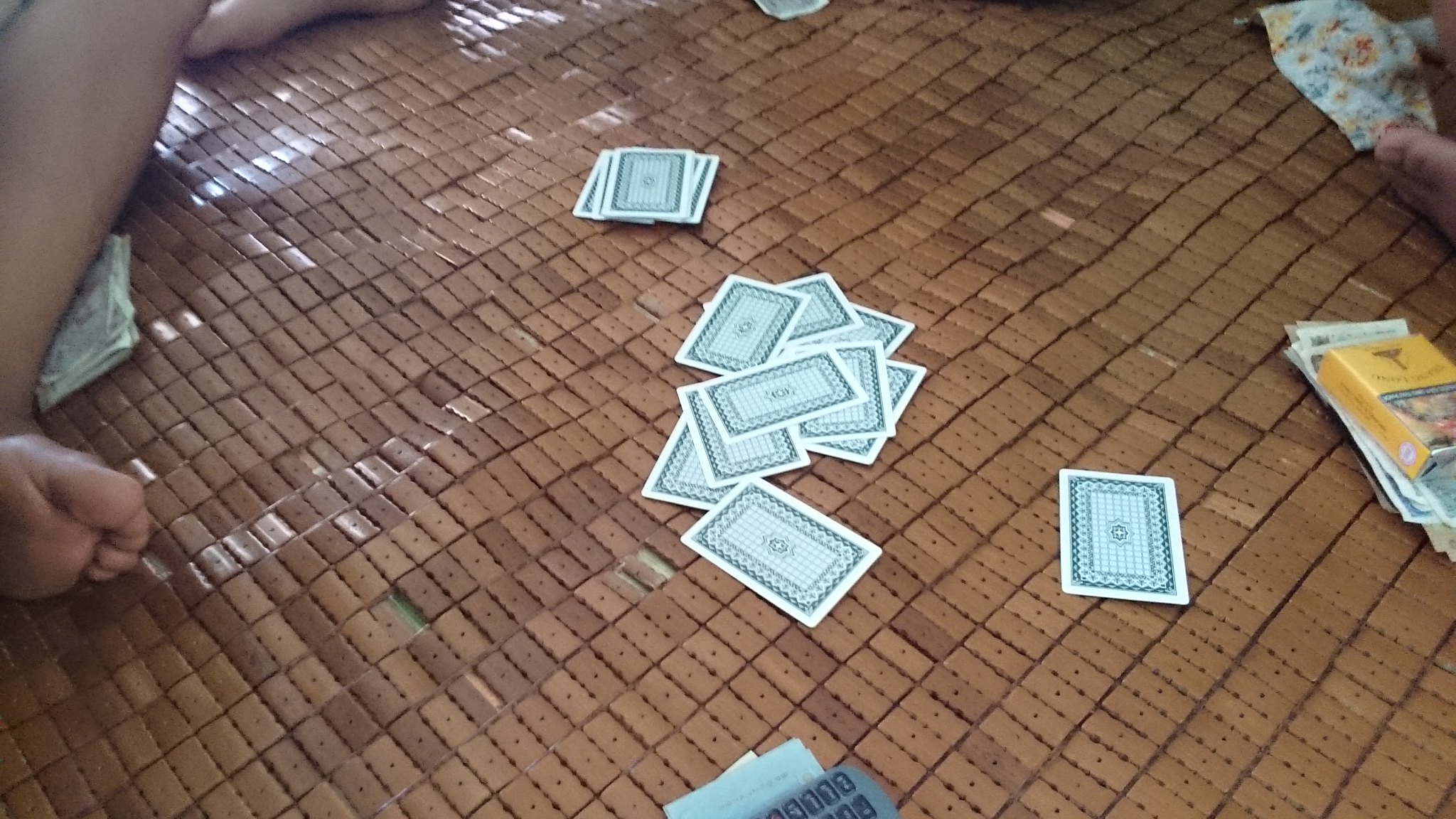The image depicts a scene of a card game in progress. In the center of the floor, a number of playing cards are arranged face down, their backs adorned with a classic pattern of green ink on a white background. To the left of the image, one can see the front of a person's shin and the top of their foot, indicating their seated position on the ground, possibly preparing for or engaging in the game. The floor below appears to be a tiled mat, consisting of small, connected brown squares.

On the right side of the photo, there is a box, potentially the original container for the deck of cards, or it could be a pack of cigarettes. There seems to be some money placed underneath this box. Furthermore, additional currency is visible beneath the person's shin on the left side of the image, suggesting that the card game involves betting. 

The arrangement of the cards in the middle of the floor includes a small pile with more cards stacked just above it, indicating that the game is ongoing and participants are carefully strategizing their next moves. The entire scene is set against the backdrop of a makeshift playing surface, emphasizing the informal yet intense nature of the game.